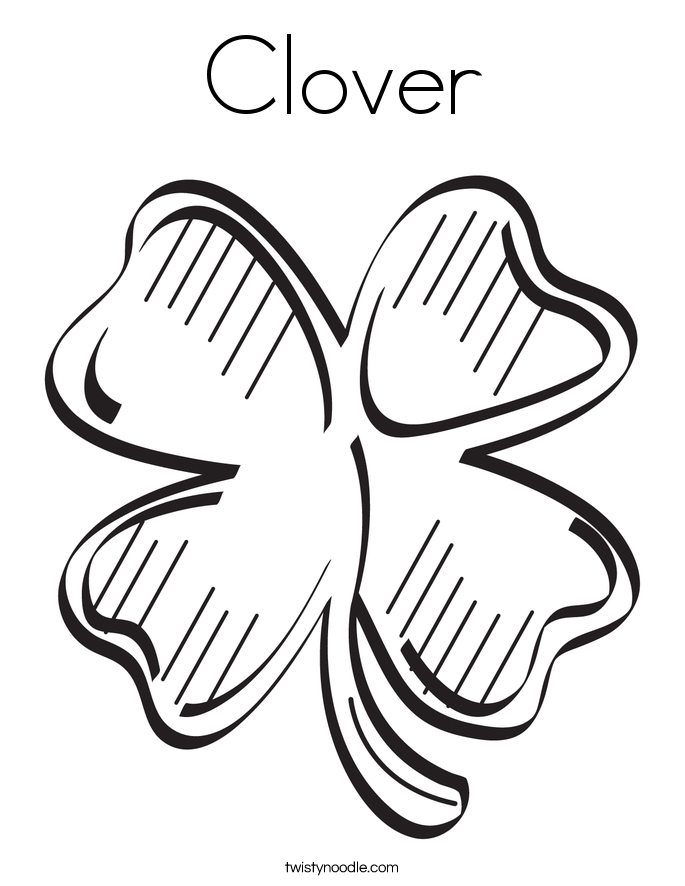This vertical black-and-white digital drawing prominently features a four-leaf clover. At the top, the word "CLOVER" is displayed in large black text. Below this, the detailed clover occupies the majority of the image. The clover itself is outlined with double black borders and is characterized by well-defined straight lines emanating from the edges of each leaf, which give it a shadow-like quality. Its stem, outlined in dark black with an internal line, is positioned towards the right. At the bottom, in very small, thin black font, is the website "twistynoodle.com," suggesting the image could be associated with the site—possibly as a logo or artwork. The entire composition is set against a plain white background, with no specific border around it, emphasizing the central clover drawing.